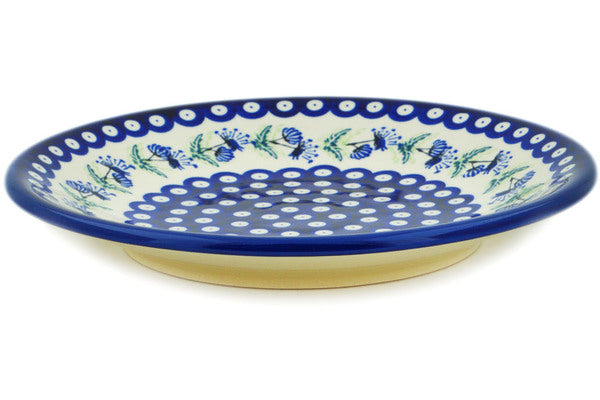This image showcases a beautifully detailed, circular ceramic plate with a glossy finish, displayed against a white background as if on a retail website. The plate's design features multiple intricate elements. The outermost border is adorned with numerous white circles, each encircled by a blue ring that forms a subtle wave-like pattern. This is followed by an off-white section decorated with blue flowers that have green leaves and black stems, all oriented sideways in a continuous ring. The center of the plate is a striking lapis blue, filled with white circles, each containing a small blue dot, creating a visually appealing contrast. The base of the plate is ivory in color, adding a subtle touch of elegance to its overall appearance.